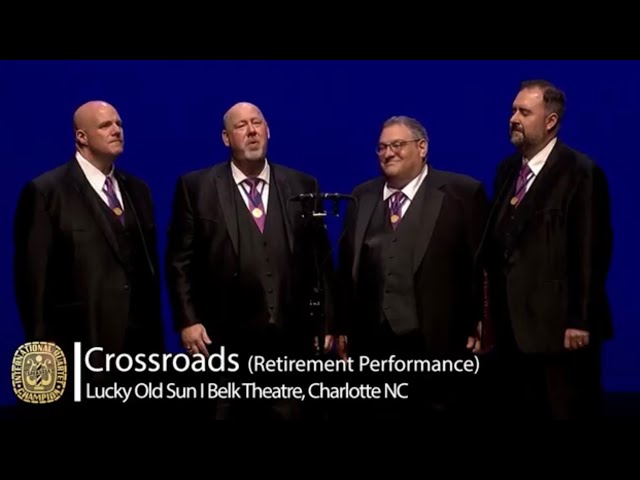The photo, seemingly taken indoors and possibly from a TV broadcast, captures a group of four men standing in front of a dark blue background. Text at the top of the image reads: "Crossroads (Retirement Performance)" and below it, "Lucky Old Sun" at Belk Theater, Charlotte, NC. 

All four men are middle to older-aged, dressed in black suits with white shirts and purple ties, and each wears a gold medallion with a purple ribbon around his neck. They appear to be gathered around a couple of microphones, likely performing. 

On the left, the first man is bald and has a straight face. Next to him, the second man, also mostly bald and bearded, seems to be singing or speaking. The third man, shorter and stouter, wears glasses and is smiling, suggesting he's in a good mood. The fourth man, taller and with darker brown hair, also appears happy and engaged. To the left of the image, an insignia reads "International Champion."